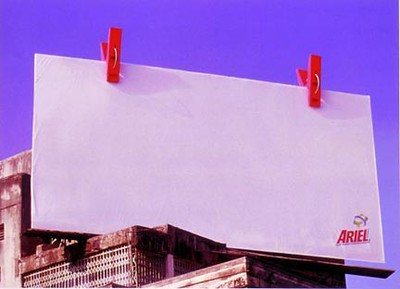The image shows an old, rickety brown building located at the bottom left corner. Atop this building sits a large, plain white billboard positioned toward the front right of the image. The billboard's fabric appears wrinkled at the top left and left side, suggesting it is being held up by two prominent red pegs or laundry clips, complete with silver wire. These clips are positioned at the top of the billboard, one on the left and one on the right. The text "ARIEL," capitalized and in bold red letters, is written prominently in the bottom right-hand corner of the billboard. The background of the image features a deep blue, almost purplish sky, creating a stark contrast with the white billboard and emphasizing its message.